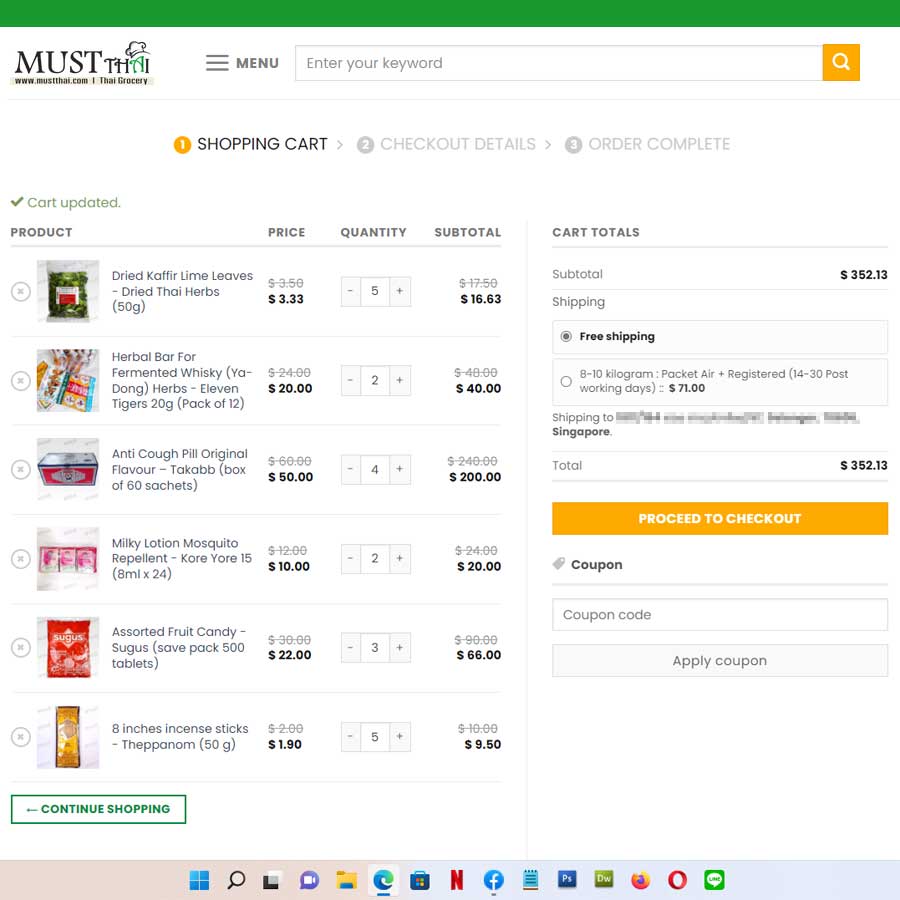This is a detailed screenshot of a desktop on a Windows device. The taskbar at the bottom features several commonly used icons, including the Windows Start button, a spotlight search icon, a webcam application, Microsoft Edge, the Microsoft Store, Netflix, Facebook, Adobe Photoshop, Mozilla Firefox, Opera browser, as well as two unidentified icons, one of which might be Adobe Dreamweaver, and another labeled "Lime."

The primary display is centered on a web browser open to a website named MustThigh, accessible via thai.com, specifically for a grocery shopping page titled "Thigh Grocery." 

The webpage shows an interactive menu with search and hamburger icons, designed for easy navigation and keyword searches. The main content visible is the user’s shopping cart, which includes detailed listings of products, prices, quantities, and subtotals, all reflecting some discounts or applied coupons.

The cart includes the following items:
1. **Dried Kaffir Lime Leaves (50 grams)**: 
   - Original price: $3.50, discounted to $3.33 
   - Quantity: 5 
   - Subtotal: Reduced from $17.50 to $16.63
2. **Herbal Bar for Fermented Whiskey, Yadong Herbs, 11 Tigers (20 grams, pack of 12)**: 
   - Original price: $24.00, discounted to $20.00 
   - Quantity: 2 
   - Subtotal: Reduced from $48.00 to $40.00
3. **Anti-Cough Pill, Original Flavor, Taqabb (Box of 60 sachets)**: 
   - Original price: $60.00, discounted to $50.00 
   - Quantity: 4 
   - Subtotal: Reduced from $240.00 to $200.00
4. **Milky Lotion Mosquito Repellent, Coriore (15.8 milliliters x 24)**: 
   - Original price: $12.00, discounted to $10.00 
   - Quantity: 2 
   - Subtotal: Reduced from $24.00 to $20.00
5. **Assorted Fruit Candy, Sugus, Safe Pack (500 tablets)**: 
   - Original price: $30.00, discounted to $22.00 
   - Quantity: 3 
   - Subtotal: Reduced from $90.00 to $66.00
6. **8-Inch Incense Sticks, Teppanam (50 grams)**: 
   - Original price: $2.00, discounted to $1.90 
   - Quantity: 5 
   - Subtotal: Reduced from $10.00 to $9.50

The cart offers options to continue shopping or proceed to checkout. The total subtotal is $352.13, with the added benefit of free shipping. Shipping options include varying weights from 8-10 kg and registered airmail, estimated at $71 for delivery within 14-30 working days. Though the user's shipping address is mostly obscured, Singapore is visible.

In summary, the user is currently using their Windows computer to order a range of Thai-themed grocery items, detailed with product descriptions, quantities, discounts, and total costs.